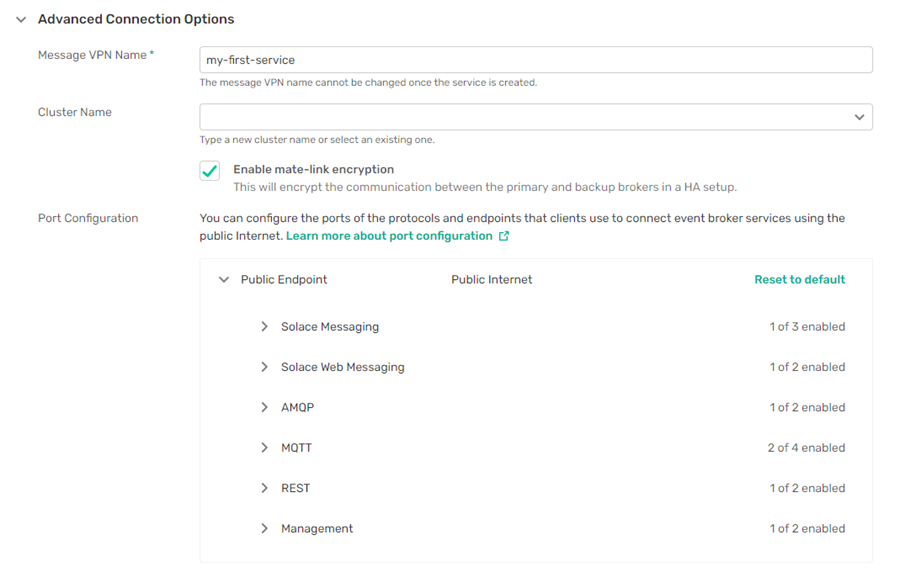**Advanced Connections Options Screen**

Displayed on a white background, this screen features the "Advanced Connections Options" section prominently in bold black text at the top. Below this title, grey text denotes the label "Message VPN Name," marked with an asterisk to signal that it is a required field. Adjacent to this label is a text box pre-filled with "My-First-Service," alongside a note stating that the message VPN name cannot be changed once the service is created.

Further down, the label "Cluster Name" appears with an empty text box featuring a drop-down menu, offering the option to either type a new cluster name or select an existing one. A blue check mark is visible next to the option "Enable Meet Link Encryption," along with a descriptive note explaining that enabling this will encrypt communication between the primary and backup brokers in the High Availability (HA) setup.

The "Port Configuration" section follows, advising users that the ports and protocol endpoints can be configured for client connections to the event broker services via the public Internet. A clickable link is provided to learn more about port configuration.

Below this, there are two buttons labeled "Provide Public Internet" and "Reset to Default."

Finally, a list of enabled services is presented, which includes:
- Solace Messaging: 1 of 3 enabled
- Solace Web Messaging: 1 of 2 enabled
- AMQP: 1 of 2 enabled
- MQTT: 2 of 4 enabled
- REST: 1 of 2 enabled
- Management: 1 of 2 enabled